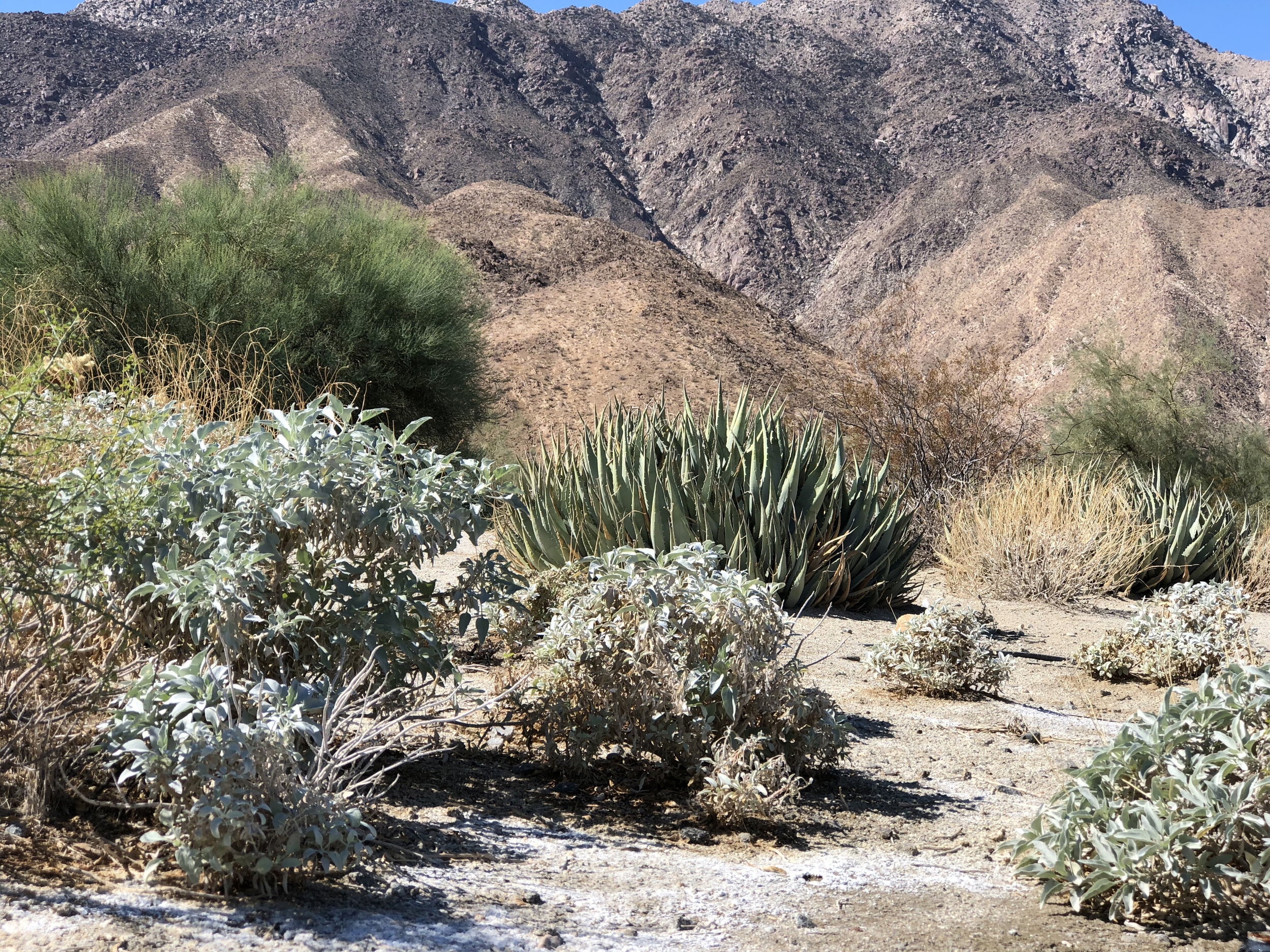This photograph captures a stark desert landscape dominated by a large mountain range that rises prominently towards the top of the image, nearly eclipsing the clear blue sky which peeks through in small areas. The desert floor is a smooth expanse of tan ground that looks flat and easy to traverse. In the foreground, the scene is dotted with a variety of spiky, cactus-like plants, small shrub-style growths, and desert foliage. These plants, ranging in height from two to three feet, display the typical pale green hues of desert vegetation. Mixed among them are rough, spiky bushes and a larger green tree. The land seems dry with no water evident, embodying the quintessential desert setting. The photograph appears to be taken around noon, indicated by the shadows cast. This scenic desert area looks like it could be part of a trail leading up the side of the mountain, inviting exploration.